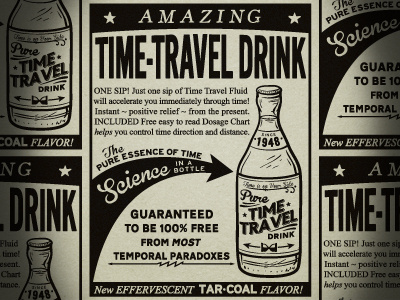The image is a black and white cartoon-style advertisement purporting to be from an old newspaper, possibly from the 1940s or 1950s, and it's a parody ad for an "Amazing Time Travel Drink." The ad is centrally displayed, flanked by partial duplications showing the top and bottom sections cut off and misaligned. At the top, there's a black bar featuring the word "AMAZING" in white uppercase letters flanked by stars. Below this, on an off-white background, bold black letters announce "TIME-DASH TRAVEL DRINK." The text below boasts that just one sip of the time travel fluid will "accelerate you immediately through time," promising "instant positive relief from the present" and a "free, easy-to-read dosage chart" that assists in controlling time direction and distance. 

An arching black arrow points from the left towards a clear bottle labeled "SINCE 1948" and proudly states, "THE PURE ESSENCE OF TIME," with the words "SCIENCE IN A BOTTLE" inside the arrow. Below this, it guarantees to be "100% FREE FROM MOST TEMPORAL PARADOXES." The bottle itself is illustrated clearly, showing the label "PURE TIME TRAVEL DRINK" warped slightly, with an hourglass icon indicating bi-directional time travel. The bottom of the ad features a black bar announcing in bold, uppercase letters, "NEW EFFERVESCENT TAR DOT COAL FLAVOR!" This advertisement, brimming with tongue-in-cheek humor, exudes a vintage charm reminiscent of mid-20th-century print media.